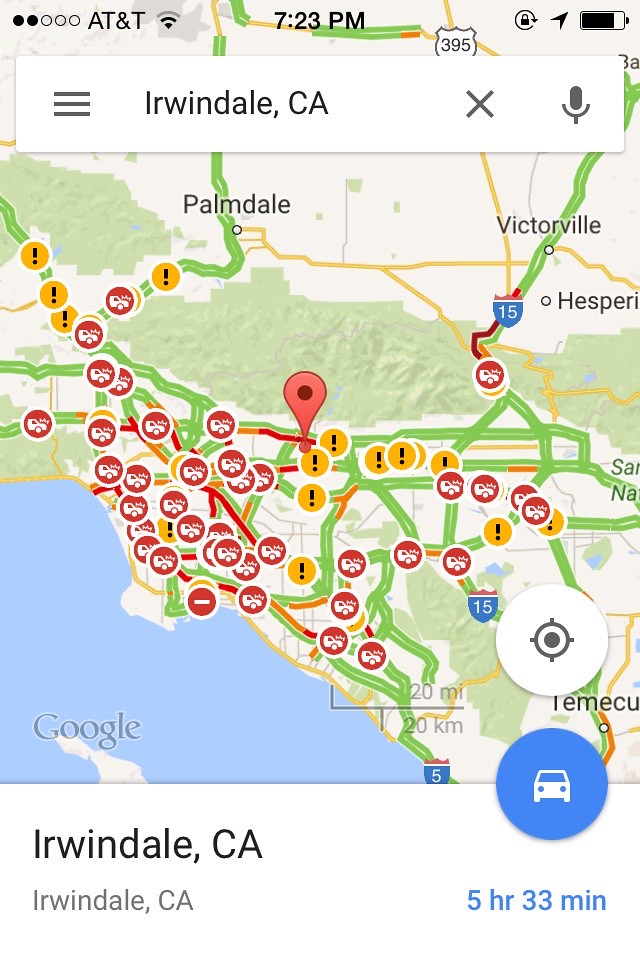The image is a detailed screenshot from Google's map app displayed on a smartphone. At the top of the screen, the status bar shows AT&T as the carrier, the time as 7:23 PM, and icons for signal strength, Wi-Fi, and battery life. Below this, a search bar reads "Irwindale, California," with an X and a microphone icon to the right. 

The main part of the image is a map centered on Irwindale, California, displaying numerous traffic symbols. The landmarks and areas on the map are dotted with yellow circles containing black exclamation points, signifying warnings or alerts, and red circles with partial images of vehicles, indicating traffic incidents or congestion. 

At the bottom of the screen, the text "Irwindale, California" appears again, along with a blue circle featuring a car icon and the text "5 hours and 33 minutes" in blue, suggesting driving time. The lower-left corner displays "Google" indicating the map source. The map itself also shows areas extending to Palmdale and Victorville.